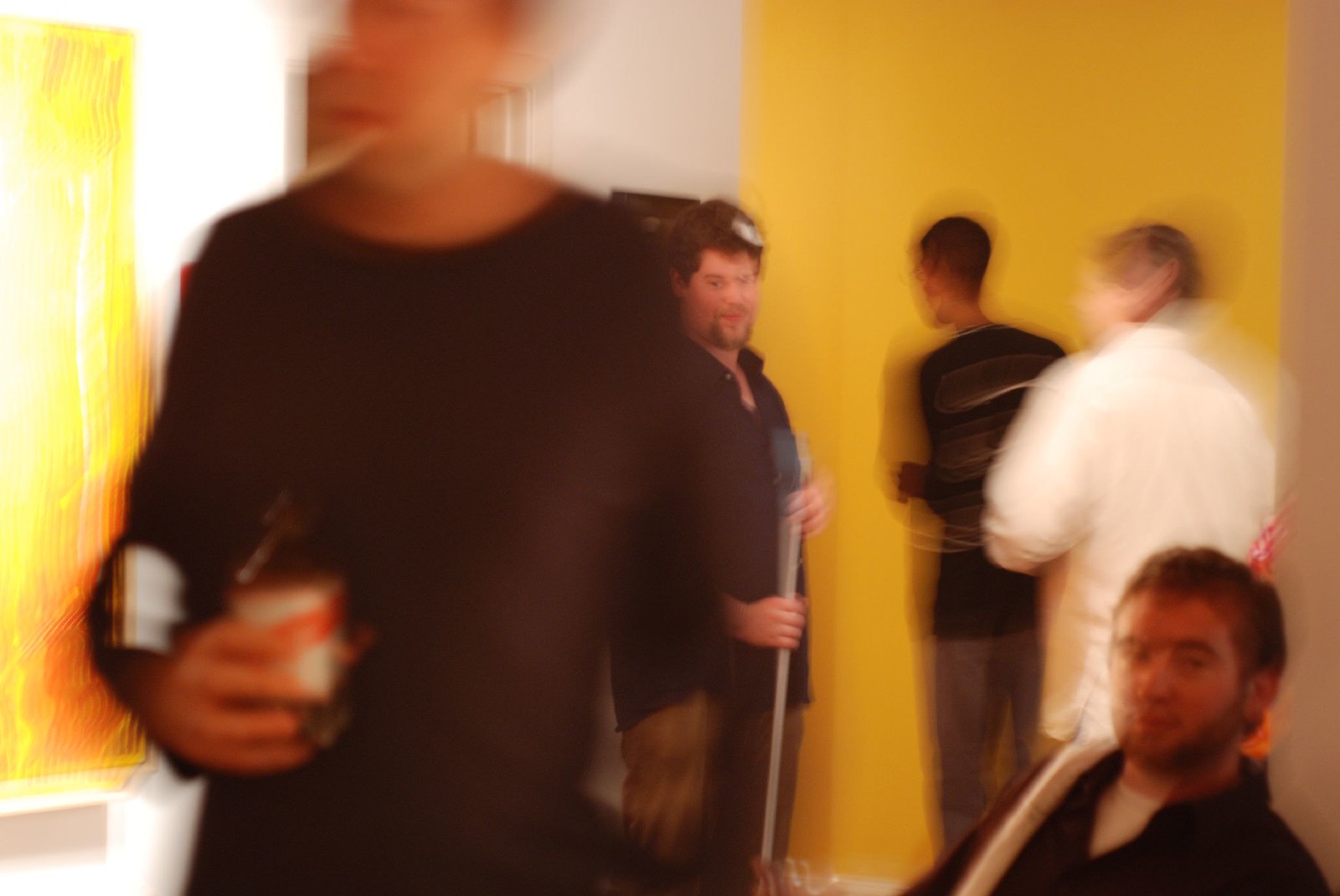This slightly blurry image captures a group of five men within what appears to be a museum setting with white and yellow walls displaying art. In the foreground, a person is seen holding a dark Lager beer in a brown bottle with a distinctive white label featuring a red bar. This individual is dressed in a long-sleeved black shirt. Behind him, a man holds what looks like a pool or broomstick. He sports a black button-down shirt that is not fully buttoned, revealing his chest, and pairs it with brown pants. He also has a goatee and brown hair with what might be a white patch caused by light reflection. 

Towards the back, a man is wearing a black sweater with gray pants. The most focused figure in the center of the image is a man in a white button-down collared shirt, holding a pool stick. Another gentleman is seated, wearing a black button-down long-sleeve shirt over a white undershirt, with his beard, goatee, and brown hair clearly visible. A white object is draped over his shoulder. This composition, despite its lack of sharpness, collectively highlights the different attires, individual features, and actions of the five men against the backdrop of the museum's artistic environment.